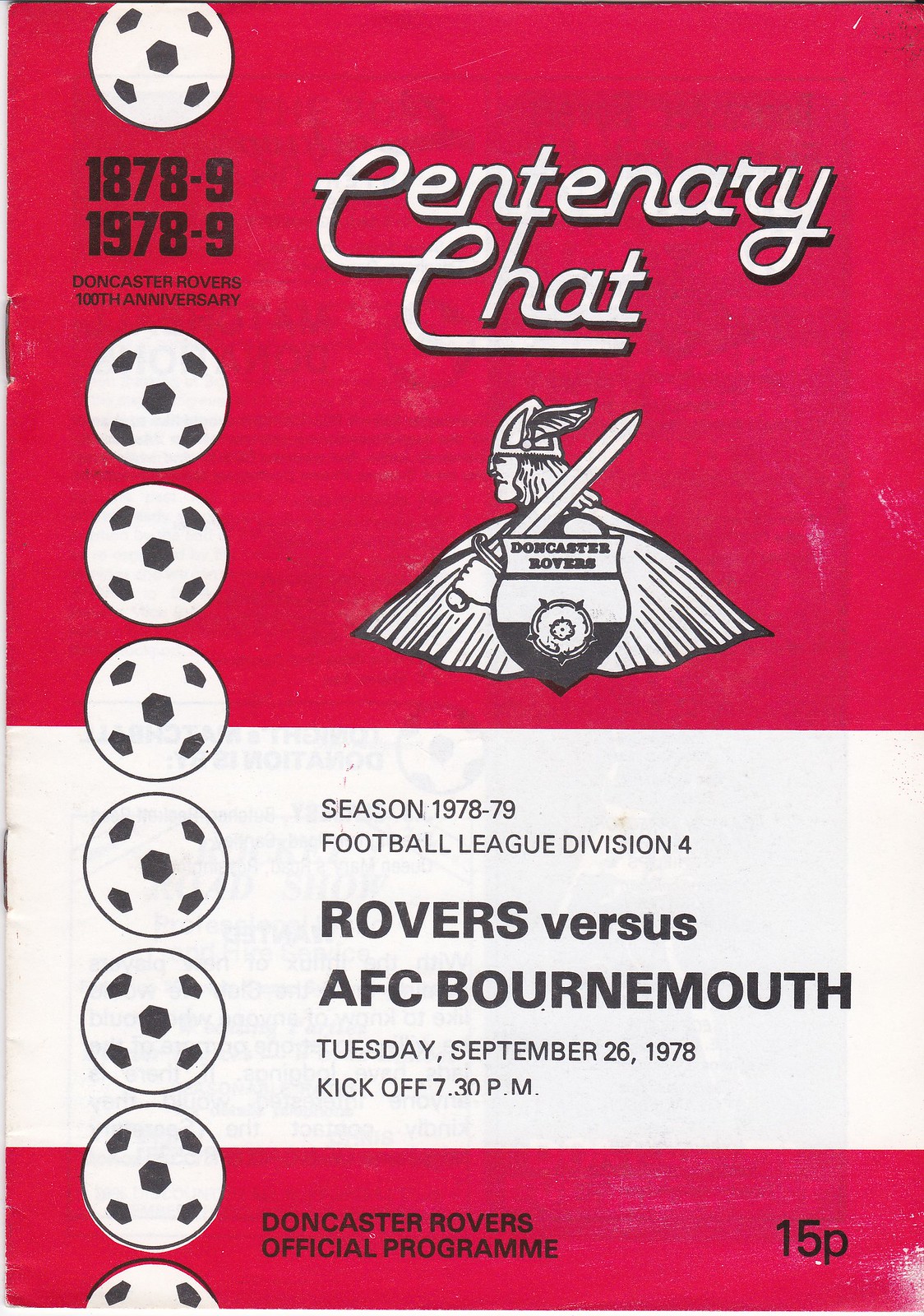This advertisement poster predominantly features a bold red background with accents of white and black. At the top, in striking white font, the title "Century Chat" is prominently displayed. Just below the title is the Doncaster Rovers logo, which depicts a knight adorned with long hair and a triangular tin helmet with a wing. The knight is equipped with a sword, a cape, and is positioned behind a shield bearing the inscription "Doncaster Rovers."

On the left side of the poster, there is a vertical column of black and white soccer balls, totaling six and a half balls. Recognized in this section is the text "1878-9 - 1978-9," emphasizing the "Doncaster Rovers 100th Anniversary."

The central part of the poster features a large white square with black text providing key information: "Season 1978-79 Football League Division IV Rovers vs. AFC Bournemouth Tuesday, September 26, 1978 Kickoff 7.30 p.m."

At the bottom, there is a prominent red stripe with black text that reads, "Doncaster Rovers Official Program 15P."

This detailed poster commemorates the Doncaster Rovers' centenary, marking a significant milestone in the club's history and promoting an upcoming match.